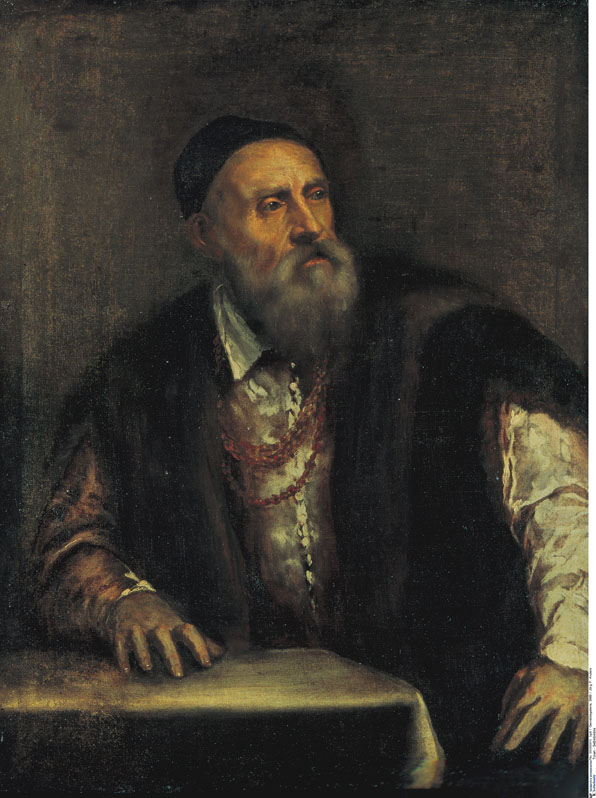This vertical, rectangular oil painting, likely from the 1600s, depicts an elderly man seated in a dark room with textured greenish-brown walls, illuminated by scattered light areas of white and yellow. The man is adorned in an elaborate outfit comprising a silky, yellowed white long-sleeve shirt beneath a thick, black fur vest that might be made from sable or ermine. His prominent gray beard and mustache, streaked with light and dark grays, frame his solemn face. On his head, he wears a small black hat or skullcap that aligns with the fur vest, suggesting a cohesive attire. Around his neck, he displays a collection of reddish-brown chains or necklaces, possibly rosary beads, hinting at a religious background. His right arm rests on his knee while his left arm is positioned on a table beside him. The table in front of him is draped with a yellowish, white cloth, standing out against the otherwise dark and muted setting. The man's contemplative gaze is directed to the viewer's left, reinforcing the portrait's deep and introspective atmosphere.